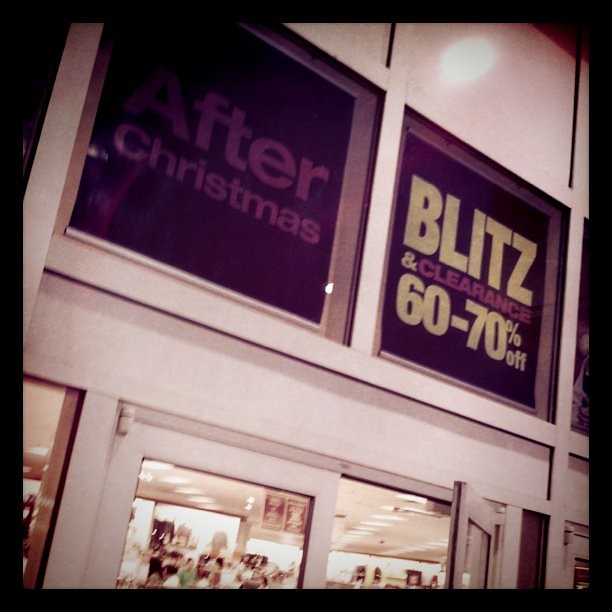A white-walled building features a dark black square on the left side, with a hint of purple tones. To the right, there's a striking yellow banner proclaiming "Texas Blitz and Clearance, 60 to 70% Off." The well-lit interior resembles a bustling department store, with shelves brimming with various items. The bright space is adorned with numerous banners and light fixtures hanging from the ceiling. A person in a green shirt is visible at the bottom, amidst the vibrant retail atmosphere, and several lamps are on display, enhancing the lively ambiance.